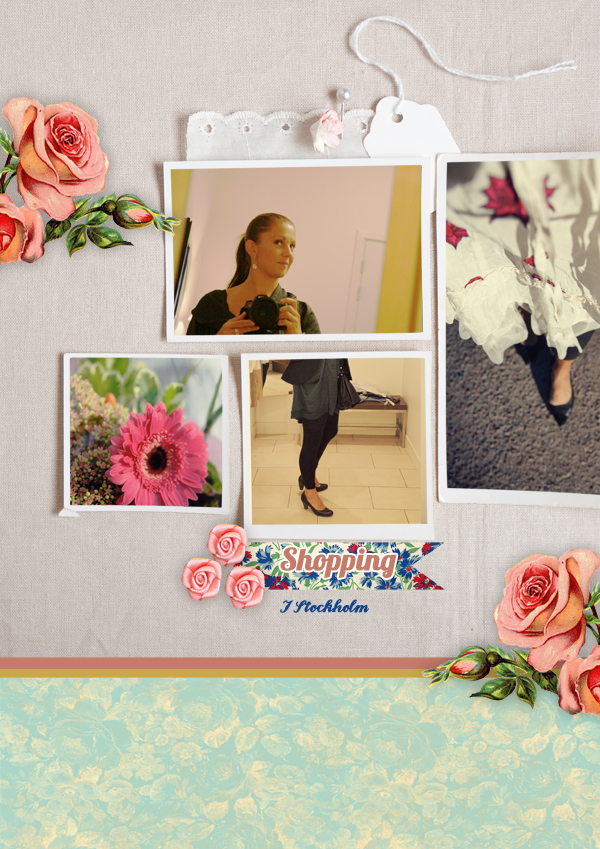The image is a detailed collage with a scrapbook aesthetic, comprising four distinct photographs of a woman and additional decorative elements. The top left photograph depicts a young woman in a black shirt with a ponytail, turned slightly to the right, against a backdrop of a white door and a yellow wall. Below this, on the left, is a vibrant pink flower with green foliage, captured in full bloom facing the viewer. On the top right, another photograph shows a woman dressed in a white dress adorned with red floral designs, standing on a gray ground with her black high-heeled foot visible. The bottom center photo highlights a pair of legs clad in black leggings, with the person wearing a black coat and black high heels, positioned on a white tile floor. A digital backdrop of white walls and pink floral decorations frames the collage, which includes playful elements like a blue floral wallpaper, lace fabric, and a white price tag. The bottom of the collage features a banner with floral motifs and cheerful text that reads, "Shopping, J. Stockholm."